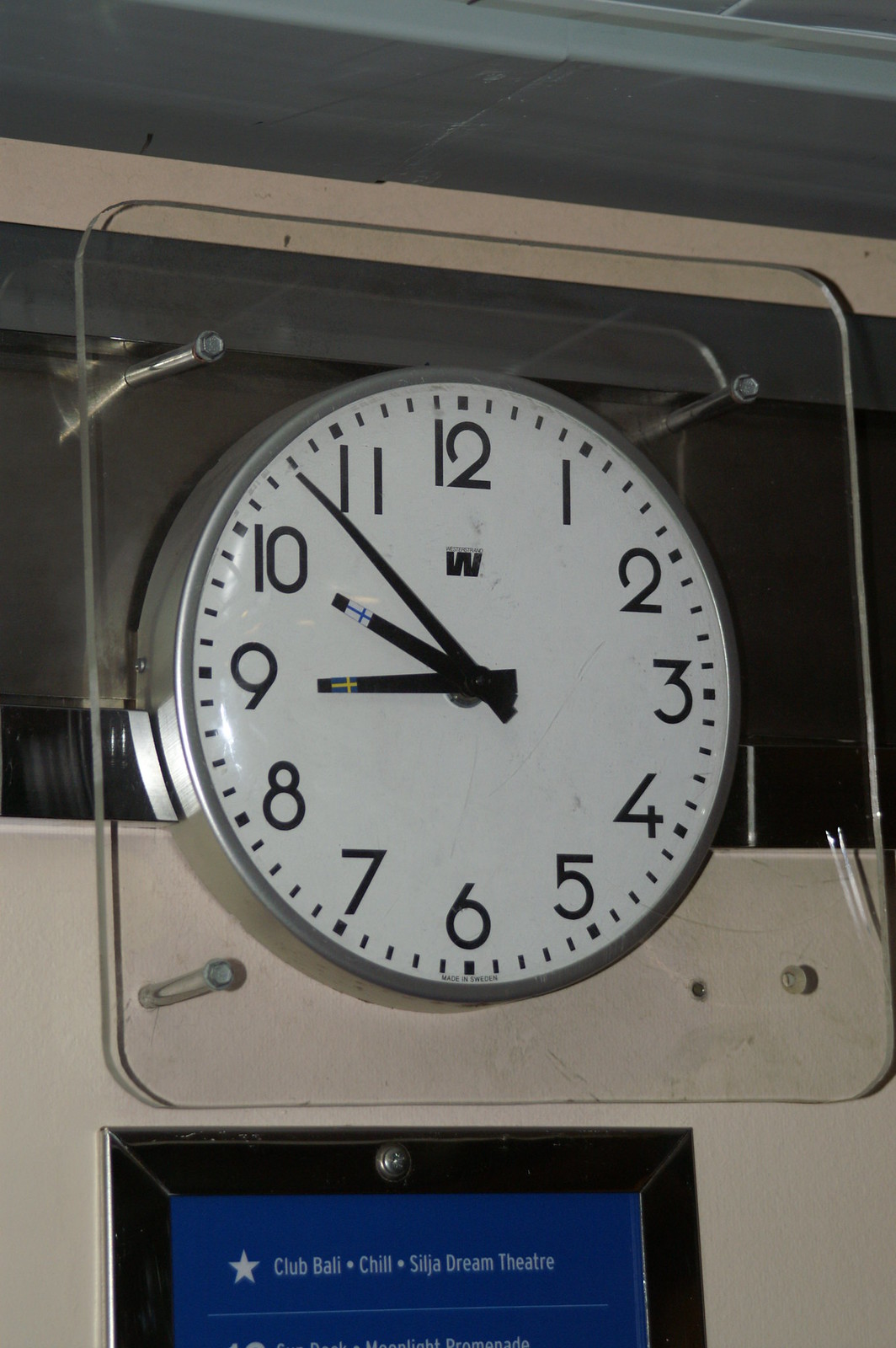A large, vintage-style clock is prominently displayed on a white wall, secured in place by a clear acrylic mount with four metal brackets. The clock's face is white with bold black numerals that evoke a 1930s-1940s font style, adding a nostalgic charm to the timepiece. It features slender black hands for seconds, minutes, and hours, all pointing to a time of 9:45. At the top of the clock face, just beneath the number 12, a giant "W" is prominently displayed, though the brand remains unidentified.

Below the clock, an electronic panel is mounted on the wall. This panel has a blue backlit screen, currently displaying the words “Club Bali Chill” followed by “Chill Something Dream Theater,” suggesting perhaps a playlist or a show schedule. This electronic screen, which seems to be integrated into the overall design of the room, adds a modern contrast to the vintage aesthetic of the clock. The lighting in the area is dim, casting soft shadows that enhance the intriguing ambiance of the setup.